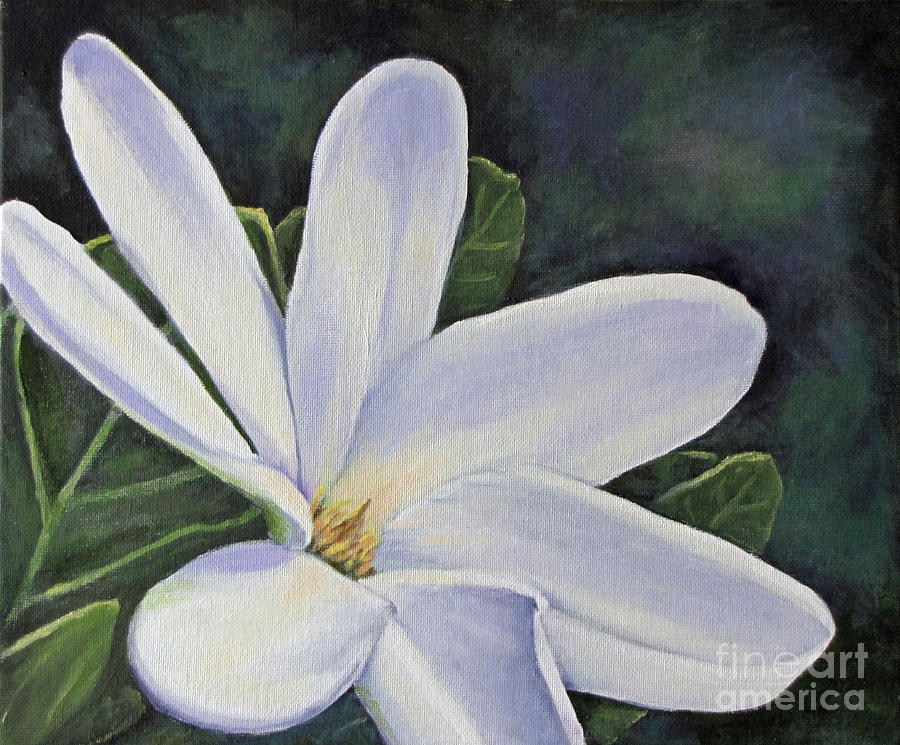This painting, done on a square canvas, vividly depicts a white flower against a dark, textured background. Rendered in either acrylic or oil paint, the flower emerges from the bottom left corner, showcasing its verdant green leaves and delicate white petals. At the heart of the flower, a mix of yellow, brown, and orange hues suggest the presence of nectar-holding flower buds. The background features swirling shades of black, dark blue, and green, applied in a circular motion, adding depth and contrast to the composition. The painting is unmarked except for a watermark in the bottom right corner, reading "Fine Arts America." The color palette spans green, white, yellow, brown, orange, black, and dark blue, creating a balanced and dynamic visual effect.